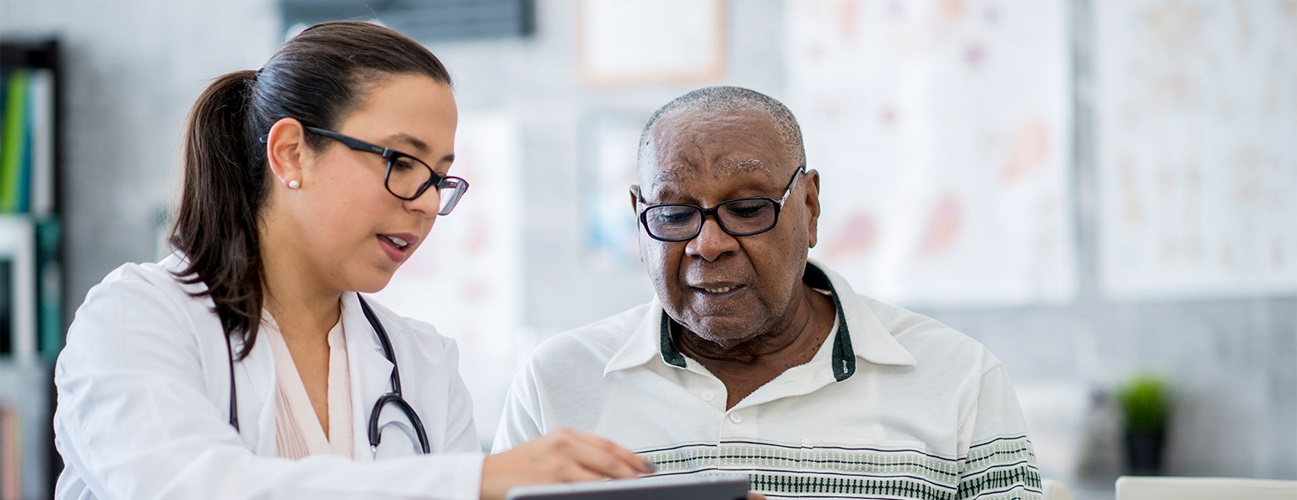In the image, a middle-aged woman, identifiable as a doctor by her white lab coat and black stethoscope draped around her neck, is engaged in a conversation with an elderly man. The doctor, who has her dark brown hair pulled back into a ponytail and is wearing black glasses and white pearl earrings, stands on the left side of the photo. She is pointing at a piece of paper that the man is holding up in front of them, possibly explaining something medical or discussing results. The man, with short, white hair and dressed in a white and green striped polo shirt, also wears black glasses. Both are intently focused on the document. The background, out of focus but discernible, features illustrations of the human body and various images, along with some green and blue books on a bookcase, suggesting a medical or clinical setting.